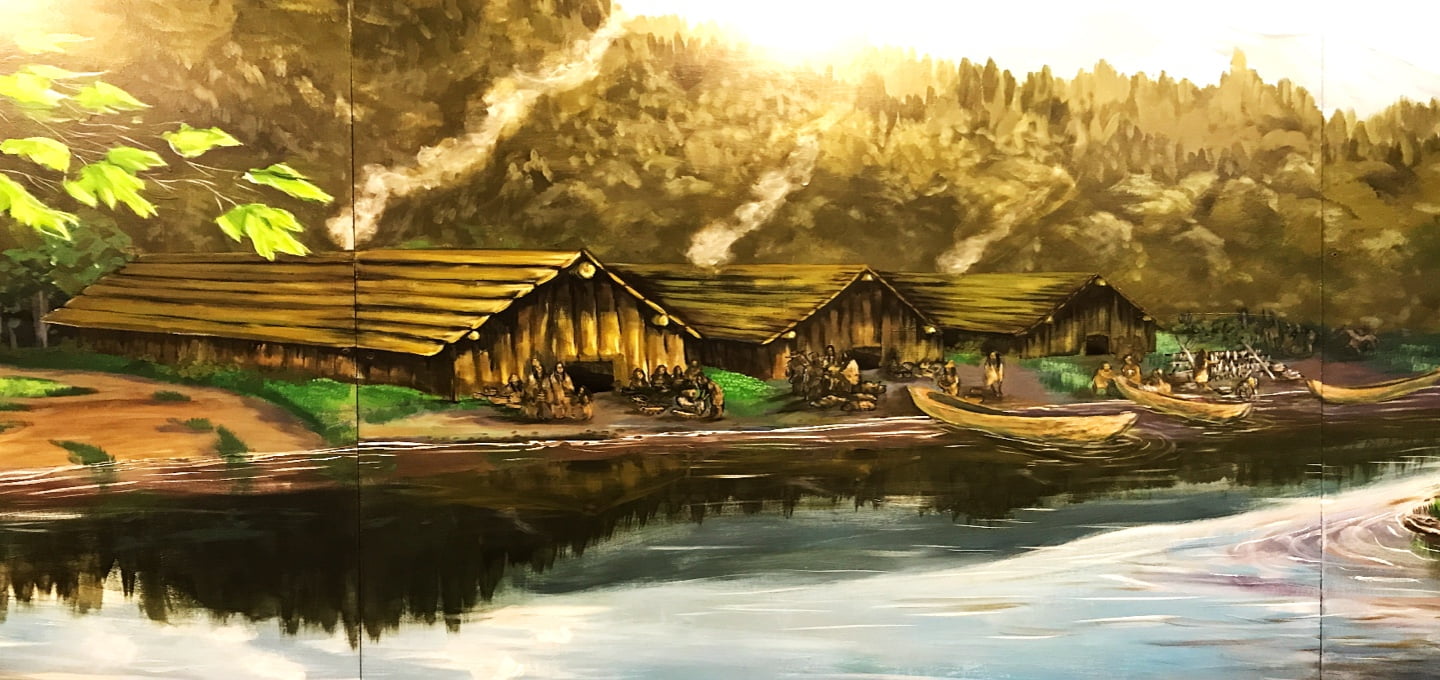The image is a detailed drawing of a serene riverside scene featuring three long wooden cabins, possibly camping cabins or part of a tribal village. The cabins are positioned along a gentle curve of a river that remains calm and reflective, mirroring the dark silhouettes of the surrounding trees and thick brush behind them. All three cabins have smokestacks with smoke curling upwards, indicating occupancy. The light source appears to be from the left, illuminating the left sides of the structures and casting darker shadows on the right. There are three canoes resting on the still water, and several people, presumably with black hair and traditional attire, are scattered around the cabins and preparing near the boats. This picturesque setting evokes a sense of simple, rustic life close to nature.